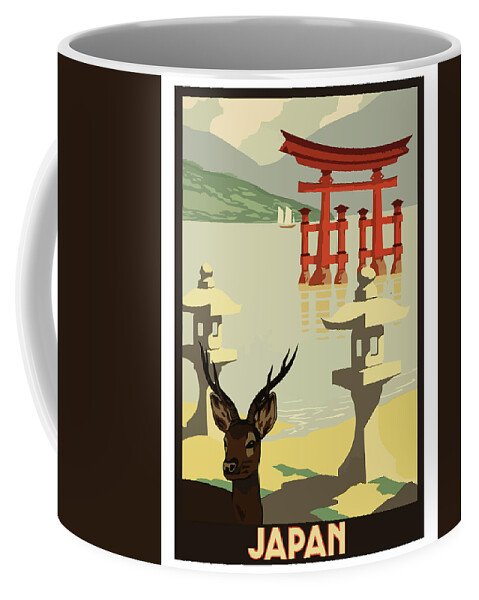The image depicts a detailed design on a ceramic coffee mug, predominantly dark brown with a curved, shiny white handle. The intricate illustration, enclosed within a vertical white rectangle on the front, showcases a serene Japanese scene. Central to the image is a brown deer with prominent antlers standing in front of a traditional red torii gate, partially submerged in a serene blue lake. Surrounding the gate are additional elements like two lantern-like structures, a sailboat with white sails, and distant green and grey mountains shrouded in mist. Below this picturesque scene, the word "Japan" is prominently displayed in yellow letters, adding to the overall Japanese theme of the mug.